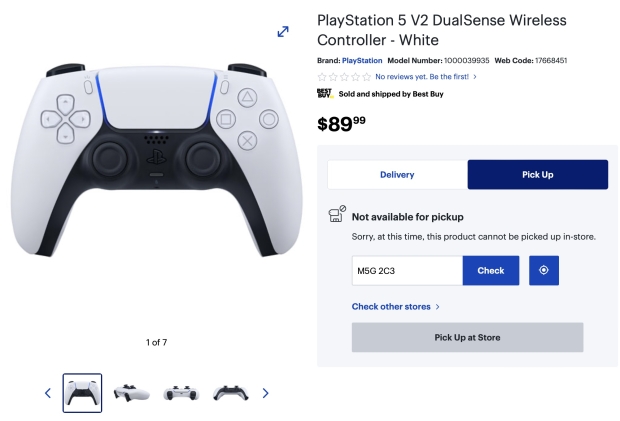The image features a PlayStation 5 V2 DualSense Wireless Controller in white. The controller belongs to the PlayStation brand and is sold and shipped by Best Buy for $89.99. Notably, the product is currently not available for in-store pickup, as indicated by the message: "Sorry, at this time this product cannot be picked up in store. Check other stores." The webpage also provides options for delivery and updates on pickup status.

The controller's design includes a D-pad with directional buttons (up, down, left, right) on the left side. On the right side, there are four iconic PlayStation buttons: a green triangle, a pink square, a blue circle, and a red X. Additionally, the controller features two analog sticks located symmetrically on the bottom left and right. This image is the first among a series of seven displayed.